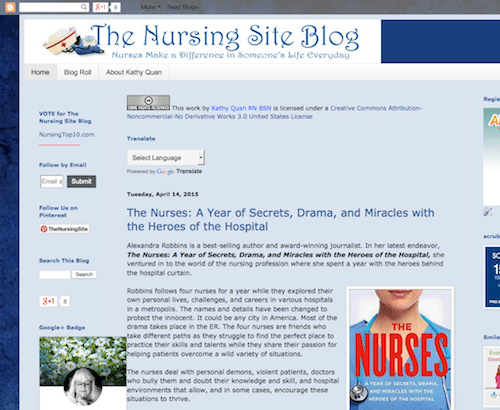Here's a cleaned-up and detailed caption for the image:

---

Screenshot of "The Nursing Site Blog" website. At the top-left corner, the title "The Nursing Site Blog" is displayed in blue font, accompanied by a small nursing hat icon. Below the header, there are three navigation tabs: "Home," "About Kathy Quan," and "Resources." The current page is set to the "Home" tab. The background under the header is light blue with a mix of blue and black text. The main article, titled "The Nurses: A Year of Secrets, Drama, and Miracles with the Heroes of the Hospitals," introduces an engaging read about the experiences of nurses. The article begins with several paragraphs in black text. There is also an image on the lower right side of the page featuring a nurse in blue scrubs with a stethoscope around her neck, with the image displaying her from the lips down to her chest. On the left side of the page, there is a sidebar containing a text input field paired with a "Submit" button, as well as a small photograph whose details are hard to discern. The overall color scheme of the blog includes white, navy blue, and a very light navy blue.

---